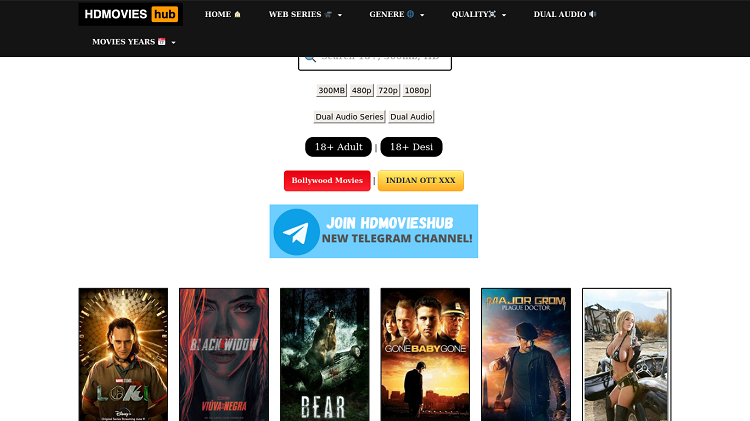The image features a website called HD Movies Hub, which allows users to download movies from various categories and in different file qualities. Along the top of the site, there is a grey rectangle that includes the logo "Red HD Movies" on the top left corner. Next to the logo, there are several menu options including Home, Web Series, General, Quality, Dual Audio, Movie Years, and more. In the center of the screen, there is a search bar where users can type in specific titles they are looking for, or filter content by categories like 18+ Adult, Dual Audio Series, Bollywood movies, and others.

The website provides the option to download movies in multiple resolutions, such as 300 MB, 480p, 720p, or 1080p, depending on the user's preference. Beneath the menu and the search bar, there is an example row showcasing some of the available movies including titles like "Black Widow," "The Bear," "Gone Baby Gone," and "Major Grom." The layout is user-friendly and designed to help users easily find and download their desired movies.